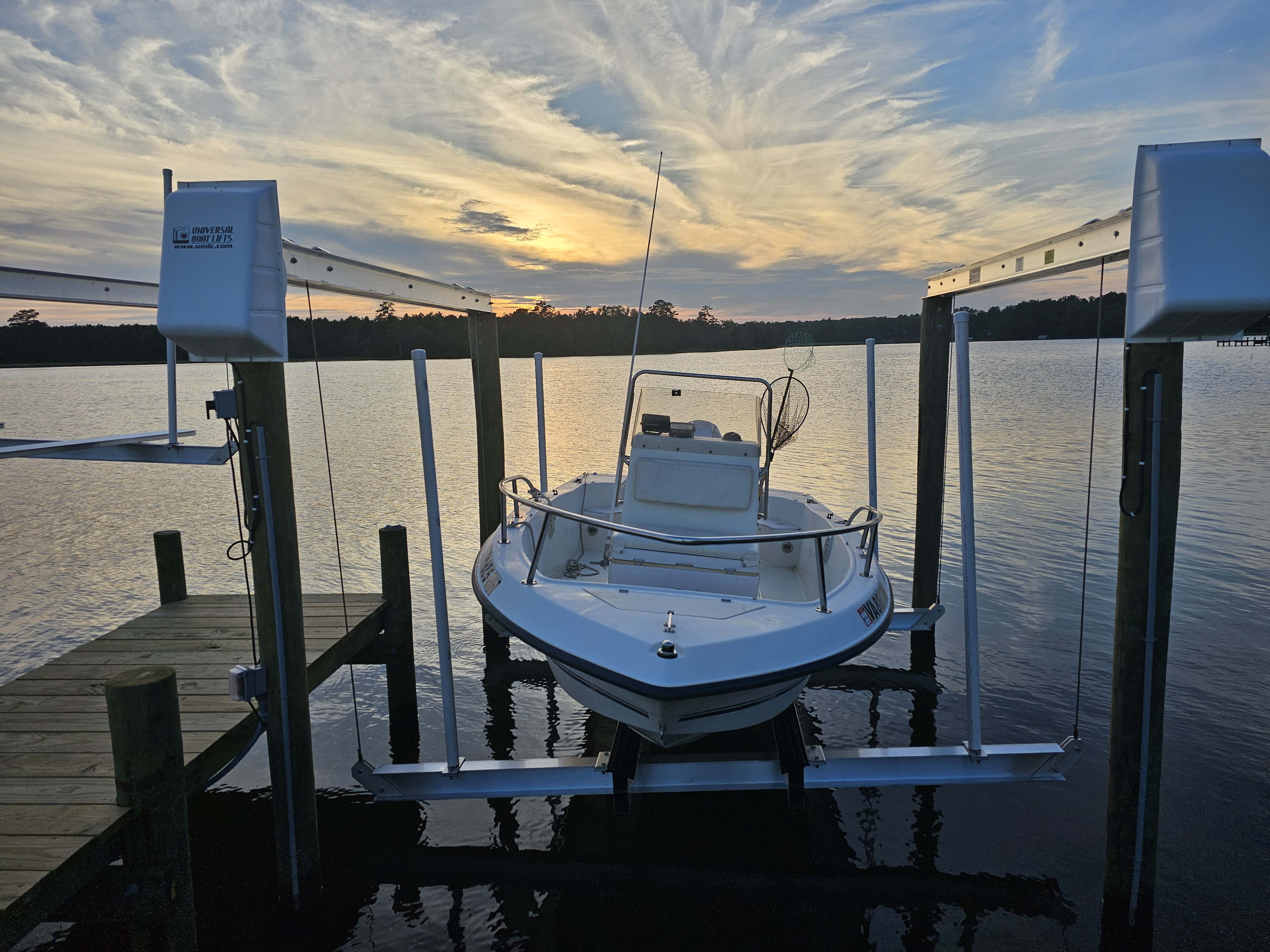This photograph captures a serene lakeside scene either during early morning or sunset. The sky is streaked with white clouds, softly illuminating the landscape. In the distance, a tree-lined land mass or possibly a small island stretches across the horizon, reflected in the dark, glistening water. To the left of the frame is a brown wooden dock with four visible suspension logs. On this dock sits a white speedboat, still hoisted above the water on metal rails by a machine designed for boat handling. This setup casts subtle shadows on the lake's surface. The boat, featuring an aluminum guard rail, awaits its descent into the water, perfectly poised against the backdrop of the tranquil, cloud-streaked sky.